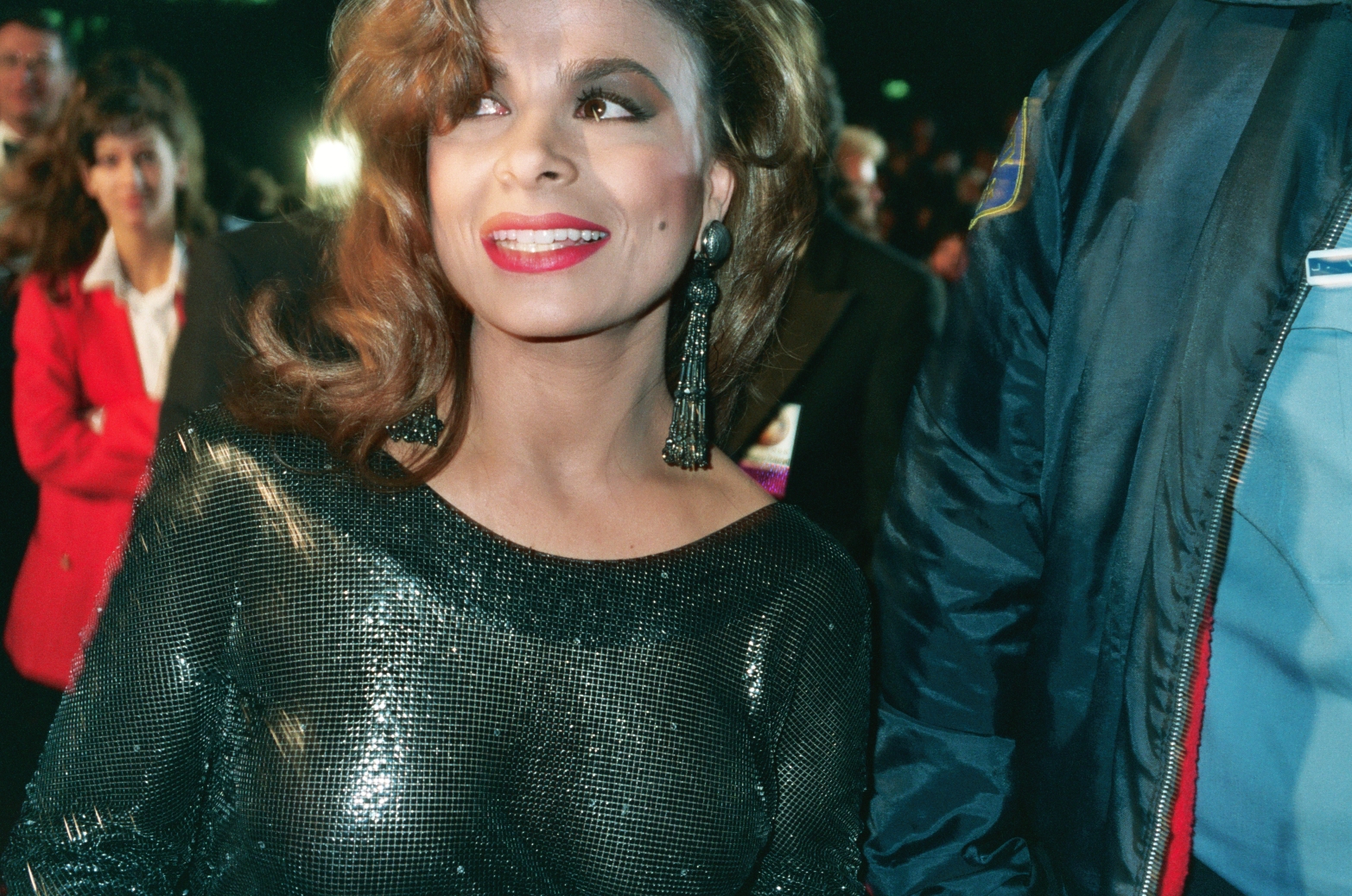The image showcases Paula Abdul, the singer, standing outside at night. She is radiant, wearing a glimmery dark outfit with a semi-transparent black, metallic-material shirt. Her shiny, long, wavy brown hair frames her face, which is adorned with bright red lipstick, eye shadow, and a distinctive beauty mark on her left cheek. She completes her look with long, dangly black earrings. Paula is smiling warmly, revealing her white teeth, and casting her gaze towards the upper left corner of the photograph. Next to her stands a large security guard dressed in a blue jacket featuring a blue and yellow patch. In the background, there's a woman with long dark brown hair wearing a red jacket over a white collared shirt, as well as a man in glasses and a suit, adding to the bustling, lively atmosphere of the scene.